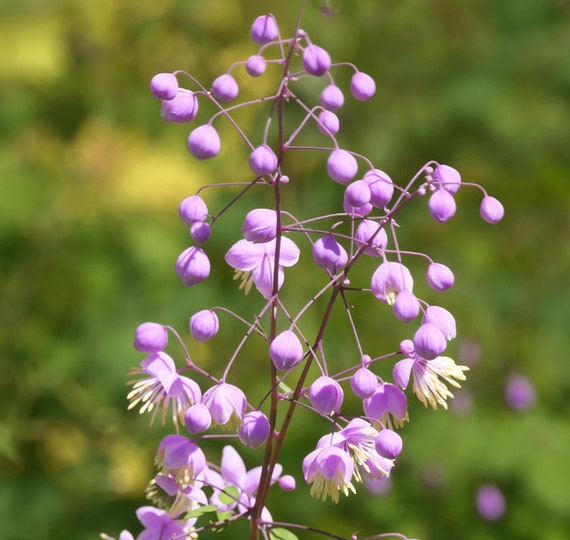This close-up image captures the delicate beauty of a Chinese meadow rue in bloom, a plant native to China. The scene focuses on the central plant, set against a backdrop of muted greens and scattered yellows, which blur into obscurity, ensuring full attention on the featured flora. The plant showcases slender, dark purple stems adorned with numerous round, purple-violet bulbs. These bulbs vary—some remain closed, while others have blossomed to reveal feathery, white protrusions tipped in yellow, reminiscent of petite fringes. At the base, small, dainty green leaves offer subtle support to the otherwise fragile, thin-stalked plant. The background hints at additional flowers, contributing to the sense of a sunlit, vibrant garden where this plant thrives.